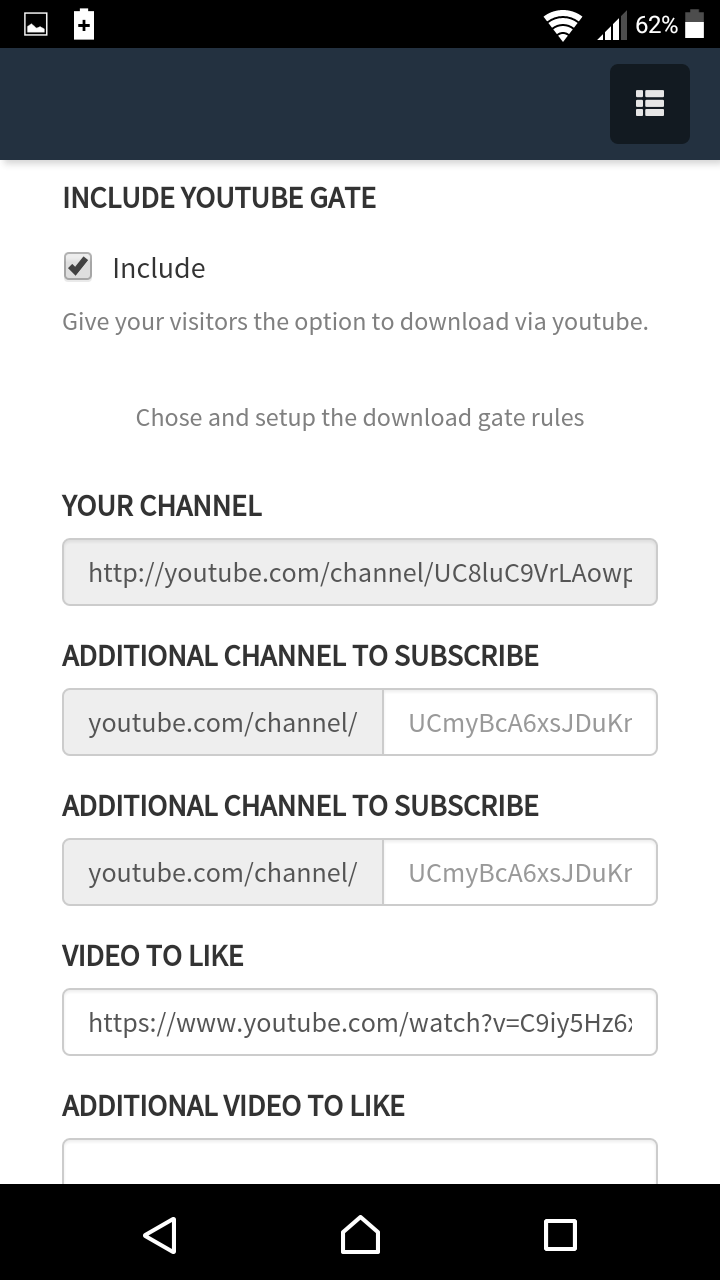The image is a vertically elongated screenshot from a cell phone, approximately two and a half times taller than it is wide. At the top 5% of the image is a black bar containing common cell phone indicators such as the battery meter and signal strength icons on the right side, and presumably some app icons on the left.

Below that is a gray bar spanning the entire width of the image, occupying about 10% of its height. In the upper right corner of this bar, there are three horizontal white lines inside a black box, which likely serves as a menu button.

The main content of the screenshot features a white background with black and gray text. At the very top of the main content, aligned to the left and in capital letters, it reads: "INCLUDE YOUTUBE GATE." Below this heading is a checkbox with a gray background and a black check mark. To the right of the checkbox is the word "Include."

Further down, there is smaller gray text that states: "Give your visitors the option to download via YouTube." After a brief gap, more gray text reads: "Choose and set up the download gate rules."

Towards the bottom of the image, bold black capitalized letters spell out: "YOUR CHANNEL," followed by a blank space.